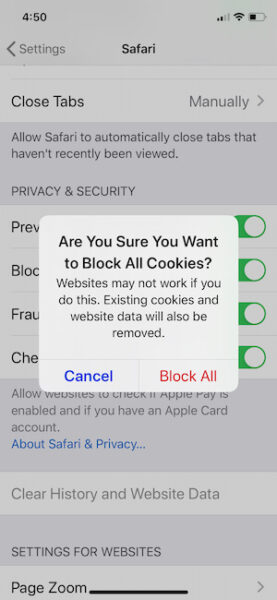The screenshot depicts the Safari settings on an iPhone, where a prominent dialog box has appeared with the message: "Are you sure you want to block all cookies? Websites may not work if you do this. Existing cookies on websites will also be removed." Below the message, there are two buttons: "Cancel," highlighted in blue, and "Block All." The dialog box covers a significant portion of the screen, but several underlying settings are still partially visible, including options such as "Close Tabs," which is set to "Manually," and other settings like "Clear History and Website Data" and "Page Zoom." The background also shows a list of toggles, the details of which are not entirely legible. This dialog serves as a warning that blocking all cookies could disrupt website functionality, potentially making some sites difficult or impossible to view.